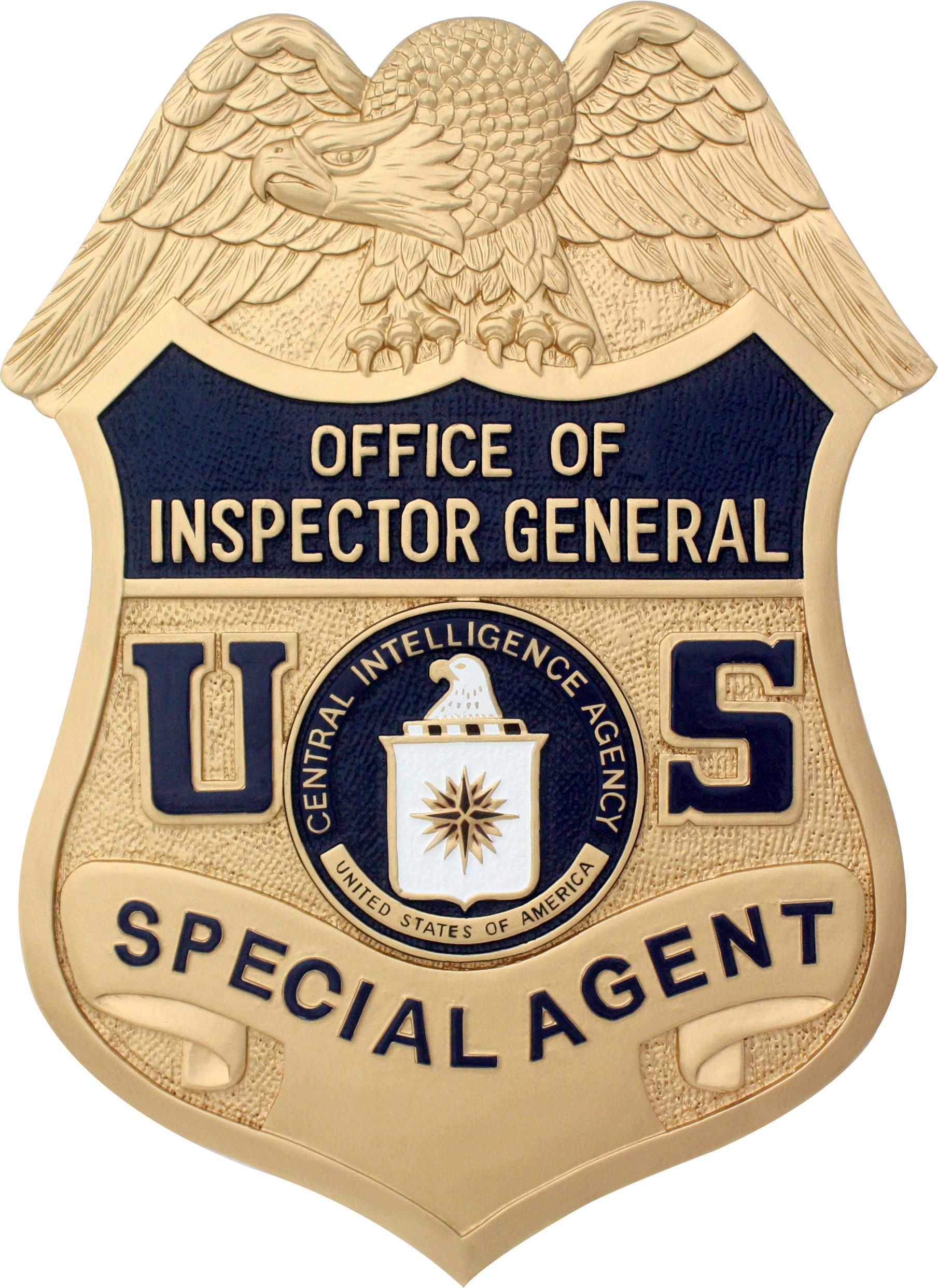The image depicts a prominent, intricately designed badge with a lustrous gold and navy color scheme against a white background. At the top, a sculpted gold eagle, facing left with its wings outstretched to the sides, appears to be perched majestically on top of the badge, forming a curved top with its wings and head. Below the eagle, a blue banner with gold lettering spells out "Office of Inspector General." Beneath this, the badge features a section with gold background and blue lettering: a "U" on the left, an "S" on the right, and a circular emblem in between. The emblem displays the text "Central Intelligence Agency, United States of America" encircling a white eagle with a flag or crest motif below it. At the very bottom, a gold banner with blue letters prominently reads "Special Agent," pointing downward to complete the shield-like contour of the badge.